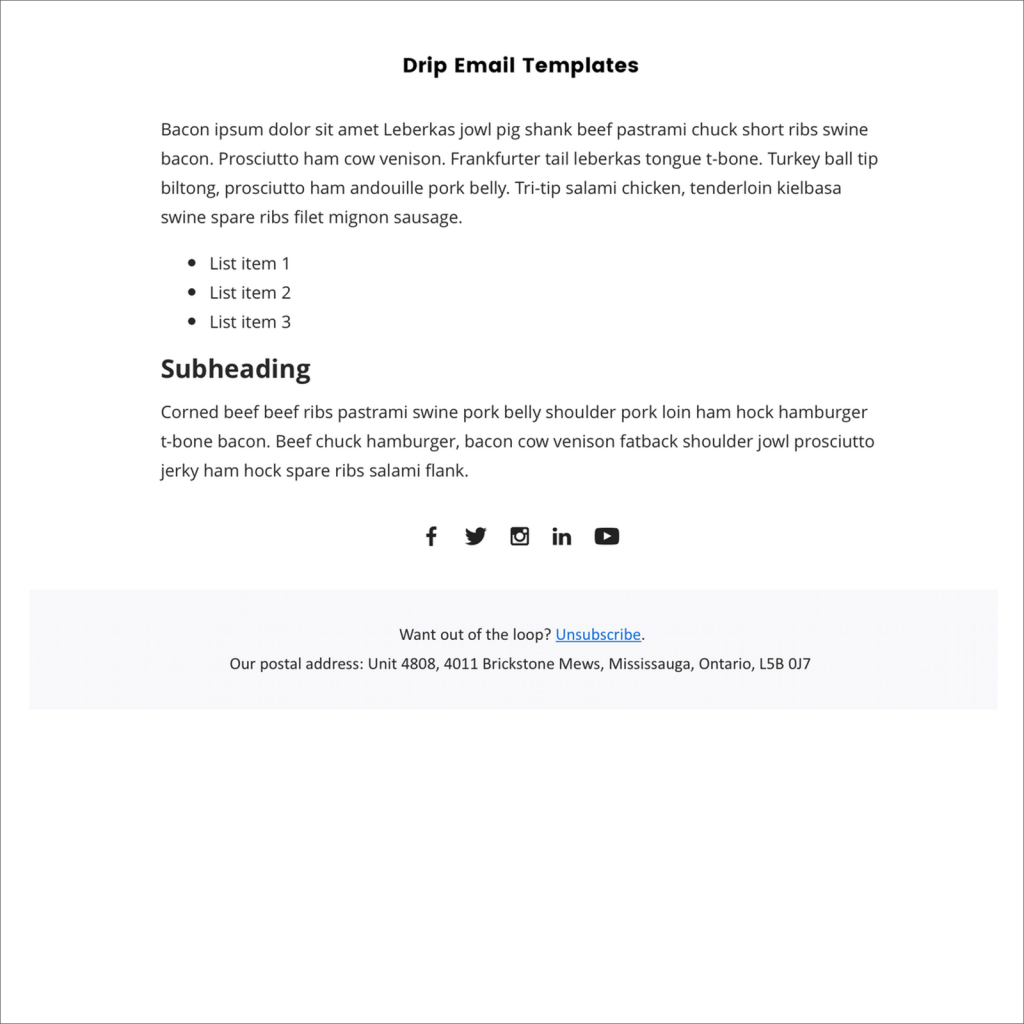In this image, we observe a webpage designed to showcase email templates. The header prominently reads "Drip Email Template." Below the title, filler text inspired by "Bacon Ipsum" occupies the space, likely acting as a placeholder. This text, a playful mix of meat-related terms, includes words like "Bacon, Ipsum, Dolor, Sit, Amet, Libercas, Jowl, Pig, Shank, Beef, Pastrami, Chuck, Short Rib, Swine, Bacon, Prosciutto, Ham, Cow, Venison, Frankfurter," and many more, forming a humorous, albeit nonsensical, passage.

Following this, there are three bullet points labeled straightforwardly as "List Item 1," "List Item 2," and "List Item 3." Beneath these points, a bolded "Subheading" is featured, emphasizing the structure of the email template. The text underneath the subheading reverts to the Bacon Ipsum theme, listing various meats such as "Corn, Beef, Ribs, Pastrami, Swine, Pork Belly, Shoulder, Loin, Ham, Hock, Hamburger, T-Bone, Bacon, Beef, Chuck, Hamburger, Bacon, Cow, Venison, Fatback, Shoulder, Jowl, Prosciutto, Jerky, Ham, Hock, Spare Ribs, Salami, Flank."

At the bottom of the page, we see icons representing various social media platforms, indicating where users can share the content or follow social media links associated with the template.